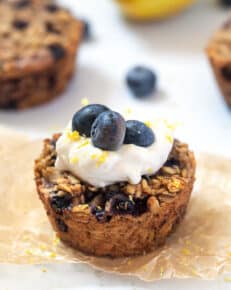The image displays a detailed photograph of a small, light brown muffin resting on a light brown, floral-patterned parchment. The muffin features specks of light yellow and black, likely indicating grains or cooked-in blueberries. It is topped with a dollop of white cream cheese frosting, adorned with three fresh blueberries and a scattering of white sprinkles and lemon zest. In the background, out of focus, are additional muffins with visible blueberry specks and a solitary blueberry on a white surface. At the top right corner, a portion of another muffin and a hint of something yellow hanging down are visible, adding depth to the composition.